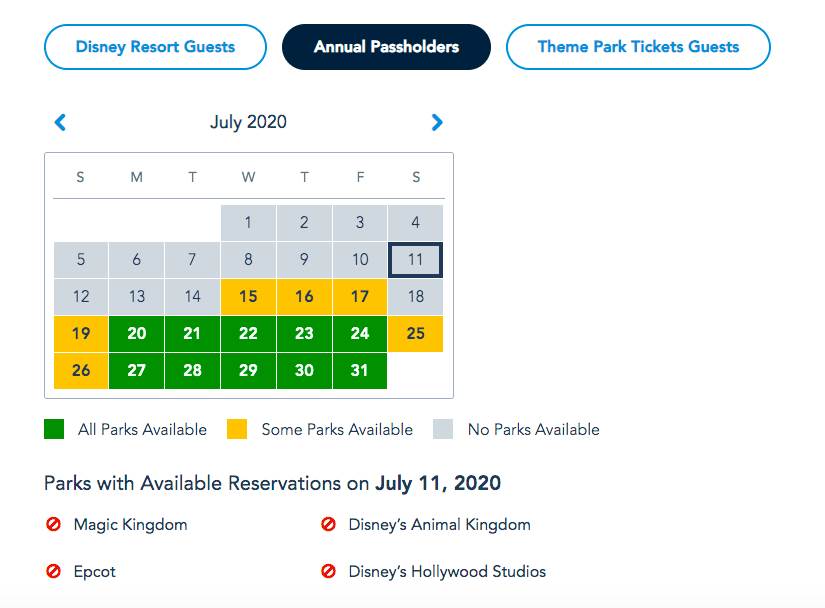In the image, there are three circles arranged from left to right against a white background. The first circle on the left is blue, with the text "Disney Resort Guests" written in blue. The second circle, to its right, is navy blue and contains the white text "Annual Passholders." Finally, the third circle is plain with the text "Theme Park Ticket Guests."

Below these circles, the date "July 2020" is displayed prominently with a left arrow on its left and a right arrow on its right, indicating navigation options for the calendar. The calendar below is structured with the week starting from Sunday and ending on Saturday. 

Notably, the first of July, a Wednesday, is in a gray box. The 11th of July, a Saturday, is outlined in a bold black box. Multiple dates including the 15th, 16th, 17th, 19th, 25th, and 26th are highlighted in yellow, suggesting limited park availability based on the legend below. From the 20th through the 31st of July, the dates are highlighted in green, indicating that all parks are available.

At the bottom, a note reads "Parks with Available Reservations on July 11, 2020." Following this note, all four Disney parks—Magic Kingdom, Epcot, Disney's Animal Kingdom, and Disney's Hollywood Studios—are each tagged with a red circle crossed out, indicating no available reservations at any of these parks on that date.